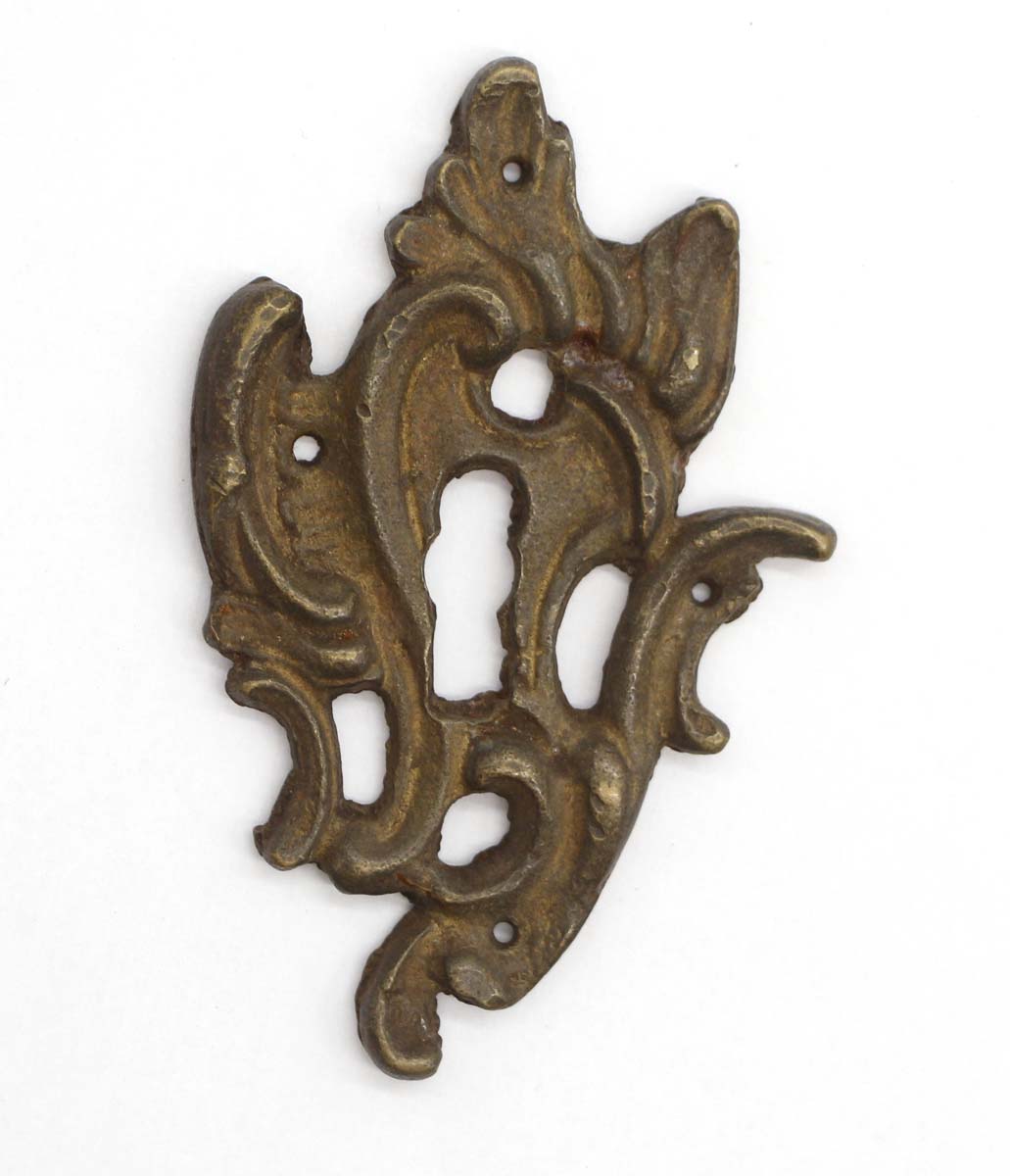This image depicts a tarnished metallic decorative piece that was once possibly brass or bronze, now showing brown, rust, and tan hues. It features a classic skeleton keyhole centrally located amidst a symmetrical, ornate design reminiscent of a Fleur-de-Lys or leaf motif. The object contains four screw or anchor points for attachment, likely to a door, wall, or potentially around a light switch or doorbell. Positioned vertically against a pure white background, the piece exhibits signs of outdoor exposure, giving it a weathered, non-shiny appearance. Despite its aged condition, the intricate detailing suggests it was intended as a decorative element in home or building construction.